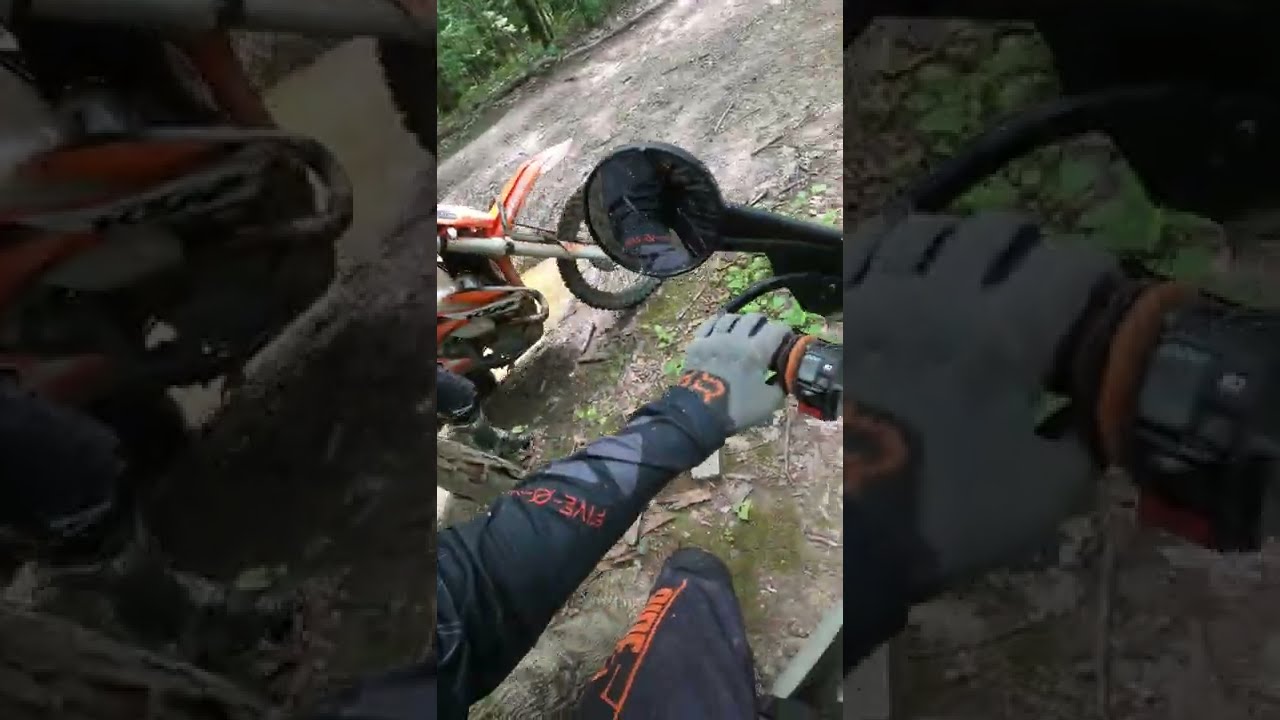The image captures a point of view from a dirt biker, highlighted by the visible left leg and arm wearing dark blue gear with distinctive orange lettering. The dirt biker's light gray glove features two orange letters, with 'R' being clearly seen as their hand grips the handlebar. Adjacent to this rider, on a red and white dirt bike, another dirt biker's right leg is also visible. The scene is set on a heavily compacted, dark grey dirt road bordered by a lush tree line in the distance. The composition of the image utilizes a split focus, with the central portion showing the full view of the dirt biker’s ride, while the left and right thirds of the image zoom in respectively on the front portion of the neighboring orange and white bike and the close-up of the gray-gloved hand on the handlebar. Both of these side panels have a darker grey filter, drawing more attention to the central action and surrounding details.